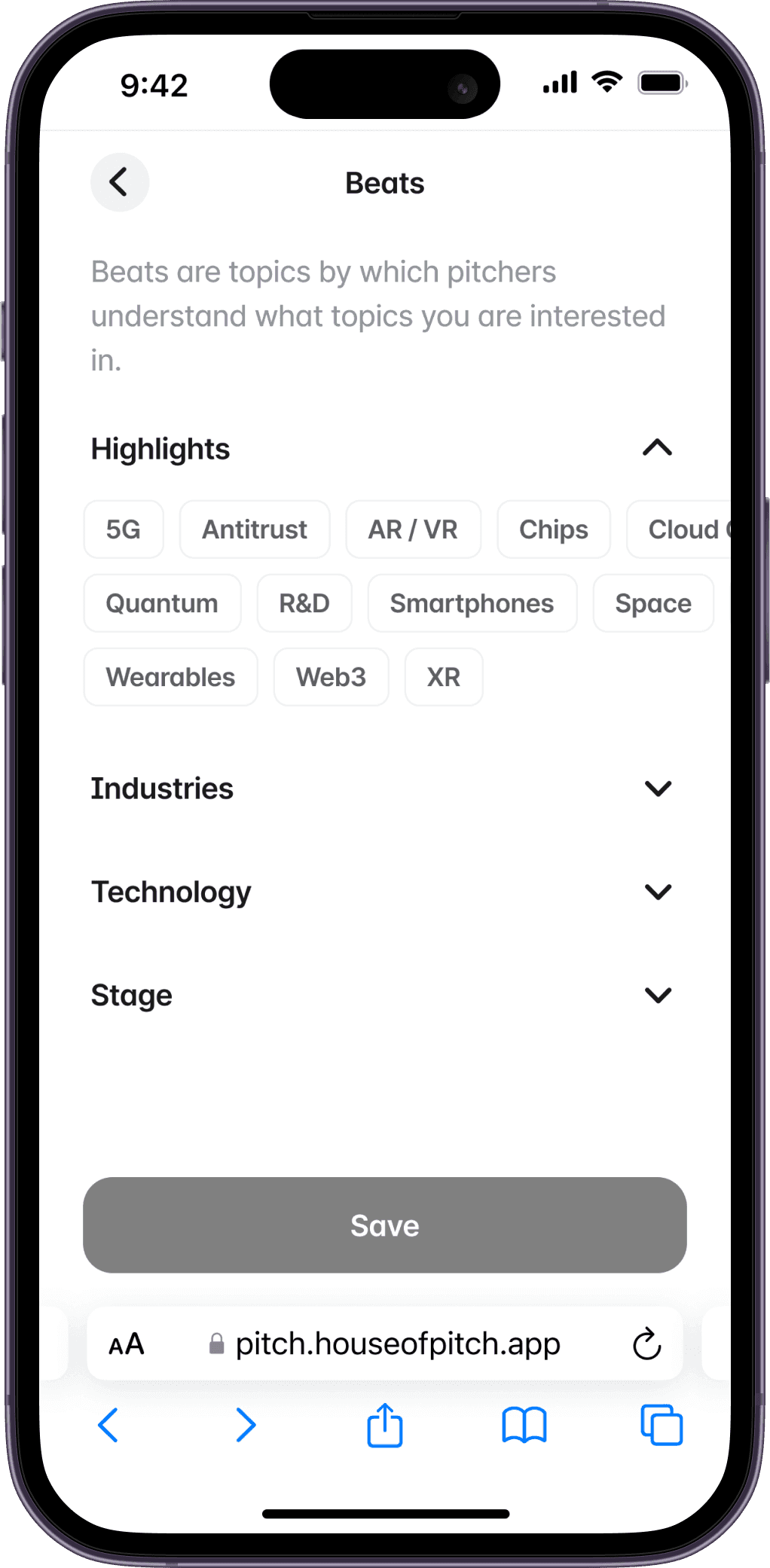The image depicts a smartphone screen displaying a web browser open to the URL pitch.houseofpitch.app. The webpage features a clean, white background with black text. At the top of the page, the word "Beats" is prominently displayed, accompanied by a black button to its left. Below this area, a descriptive text reads: "Beats are topics by which pitchers understand what topics you are interested in."

Further down, directly beneath the descriptive text, there's a drop-down menu labeled "Highlight," which has been expanded to reveal 11 options. These options include: 5G, Antitrust, AR/VR, Chips, Space, Smartphone, XR, Web 3, R&D, Quantum, and Wearables.

At the bottom of the image, there are three additional drop-down menus: "Industries," "Technology," and "Stage." Just above the URL bar at the very bottom, there is a gray button with white text that reads "Save." This button is designed to be a safe, clickable element on the page. The overall webpage layout maintains a consistent white background with black text throughout.